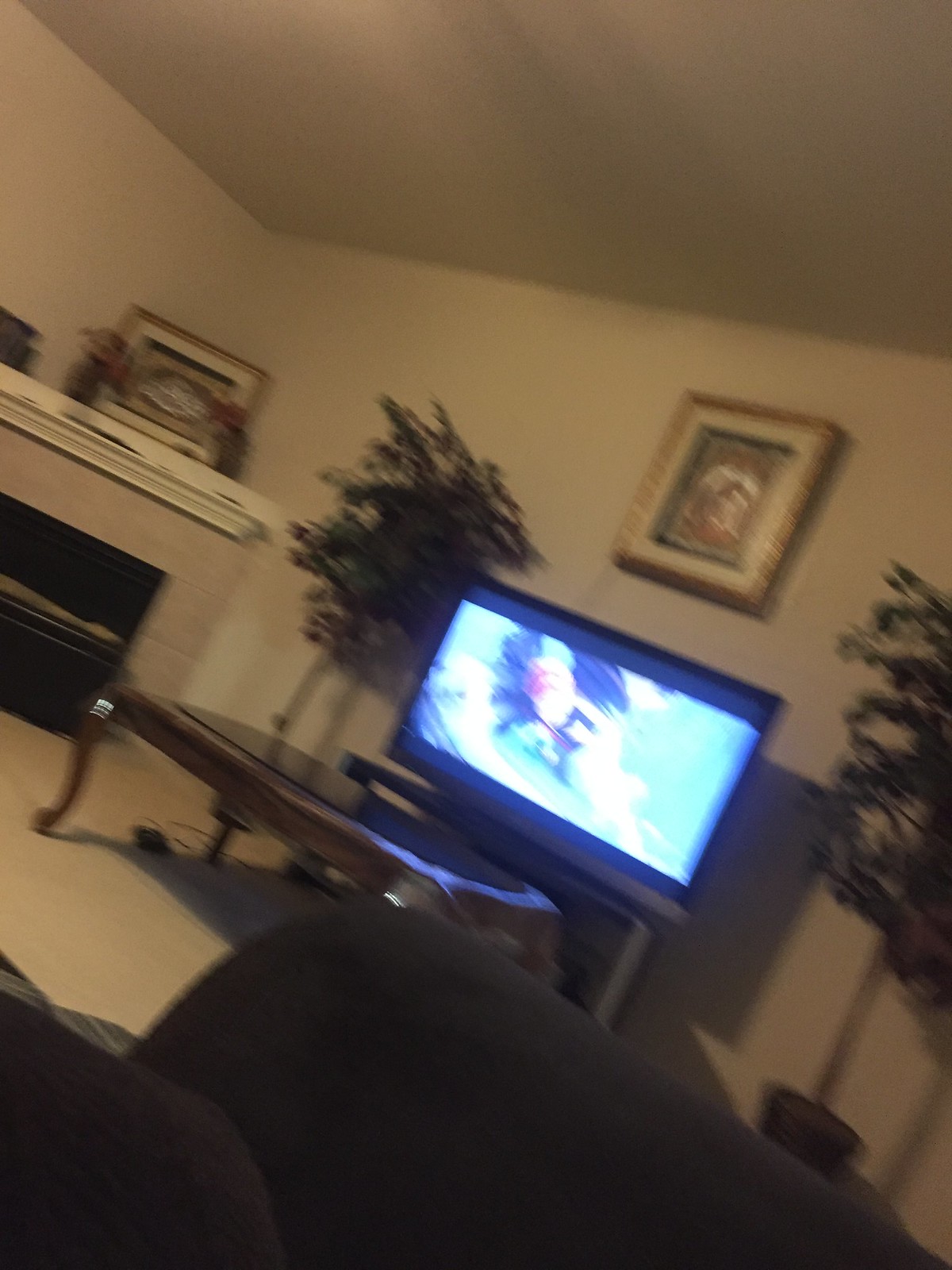This photograph, although blurry, captures the cozy and well-decorated ambiance of a living room, likely showcasing the touch of an interior designer. At the heart of the room, a wooden coffee table features a distinctive giant egg-shaped glass centerpiece. A medium-sized flat-screen TV, possibly around 32 to 40 inches, takes center stage, perched on a small entertainment stand. Directly above the TV hangs a framed art piece, while two potted plants flank the screen, adding a touch of greenery to the setup. To the left, a corner fireplace extends across two walls, adorned with flower pots and another matching framed art piece on the mantel. The room's seating arrangement includes a couch at the bottom right, partially visible with a hint of black fabric. Despite the blurriness, the attention to detail in the décor, such as the painted frames and varied textures, suggests a thoughtfully designed living space.